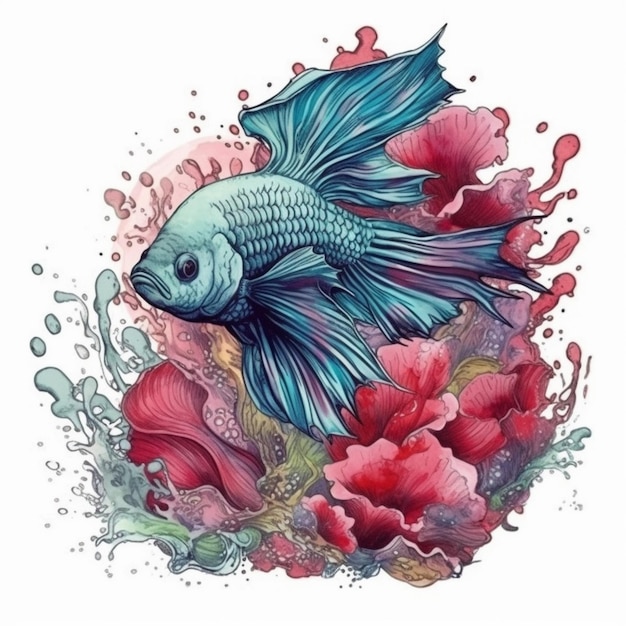This digital watercolor artwork features a blue fish facing left in a mostly profile view, adorned with long, flowing fins. The fins and tail exhibit a subtle transition to a light purplish hue, interspersed with touches of magenta. The fish is centrally placed against a white background and swims among an array of underwater flowers. These flowers, predominantly dark pink with lighter pink edges and deep pink, almost red centers, enhance the image's vibrant look. Surrounding the fish and flowers are splashes of water depicted in shades of light bluish-green at the bottom and a pinkish-red hue at the top. The water splashes create an impression of flowing motion, with scattered bubbles and smaller splashes around both the bottom and the top of the artwork, adding to the dynamic underwater scene.